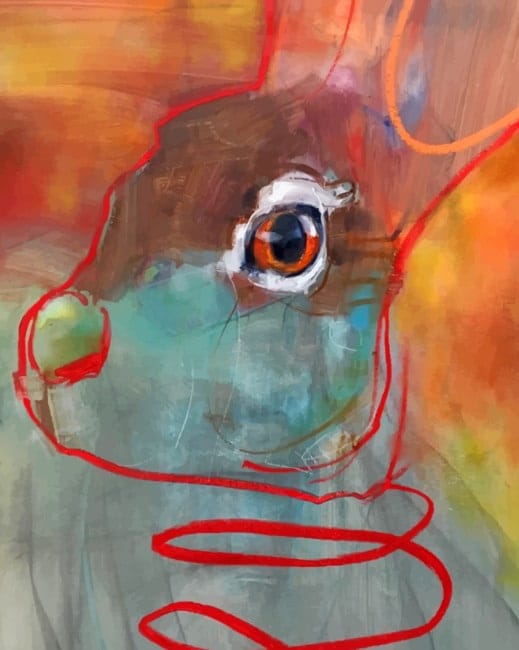This abstract watercolor painting features the head of a rabbit, prominently outlined in a red, twirly brushstroke below its neck. Its face points to the left, with an expressive, realistic eye that is orange with a distinct black pupil and white mask around it. The eye is further outlined in black. The rabbit’s head is divided into surreal sections of color: the top is brown, transitioning to a blue lower half, while the nose is strikingly green. A hint of brown can be seen below the nose, adding subtle detail. The ears of the rabbit are outlined in pink and stretch up towards the top right, beyond the frame of the image. The background of the painting is a vivid mix: pink and orange hues dominate the top, while the bottom showcases a bluish paint with hints of green. The composition is complemented by additional swirling brushstrokes extending from the neck, underscoring the abstract and surreal quality of the artwork.